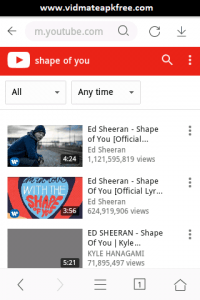This image depicts the interface of the website www.vidmateapkfree.com as viewed on a smartphone. At the top, there is a text field labeled "m.youtube.com" accompanied by a search icon, a magnifying glass, a looping arrow indicating refresh, and a downward arrow for download. Beneath this, a familiar YouTube red bar appears featuring the iconic YouTube logo within a white rectangle. In the search field below, the phrase "Shape of You" is entered.

Directly under the search field, there are drop-down menus labeled "All" and "Anytime" for sorting the search results. The page displays three video search results for the query:

1. The first result is titled "Ed Sheeran - Shape of You (Official...)" showing Ed Sheeran as the artist. It has amassed 1,121,595,819 views, and the thumbnail depicts Ed Sheeran, likely from the album cover. The video duration is 4 minutes and 24 seconds.
   
2. The second result is "Ed Sheeran - Shape of You (Official Lyrics)" and has 624,919,909 views. The duration of this video is 3 minutes and 56 seconds.

3. The third video is titled "Ed Sheeran - Shape of You | Kyle Hanagami" featuring a gray thumbnail. It has received 71,895,497 views with a runtime of 5 minutes and 21 seconds.

At the bottom of the screen are the standard navigation icons for back, forward, and home functions.